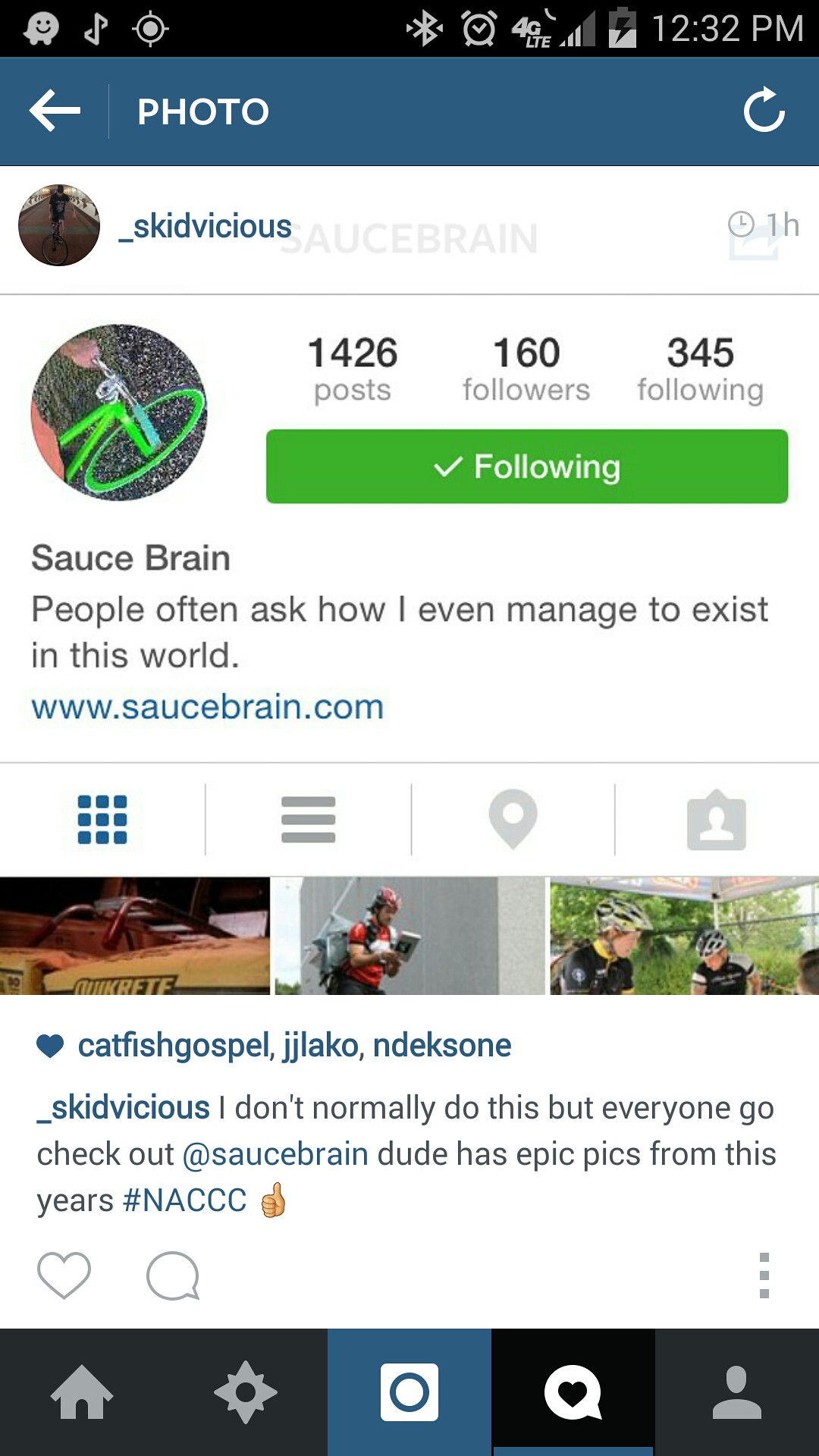The image is a detailed screenshot taken from a social media app, likely Instagram, captured on a smartphone. At the very top, there's a black status bar featuring icons for Wi-Fi, alarm, 4G, battery life, and the current time. Directly below this is a blue navigation bar with a back arrow, the word "Photo," and a refresh button.

Beneath the blue bar, the profile of the user "skydvicious" is displayed, accompanied by a small profile image. This profile shows stats including 1,426 posts, 160 followers, and 345 following. There's also a prominent green "Following" button with a checkmark indicating that the user is being followed.

The profile name reads "saucybrain," followed by a personal quote: "People often ask how I even managed to exist in this world." Below this quote, a blue-colored website link www.saucybrain.com is provided. The profile displays several images, including the front side of a green bicycle, and possibly other pictures featuring typical cycling and lifestyle moments.

At the bottom of the screenshot are additional navigation icons: a home button, a heart icon (likely for likes), and a user profile button, emphasizing the app's social interaction features.